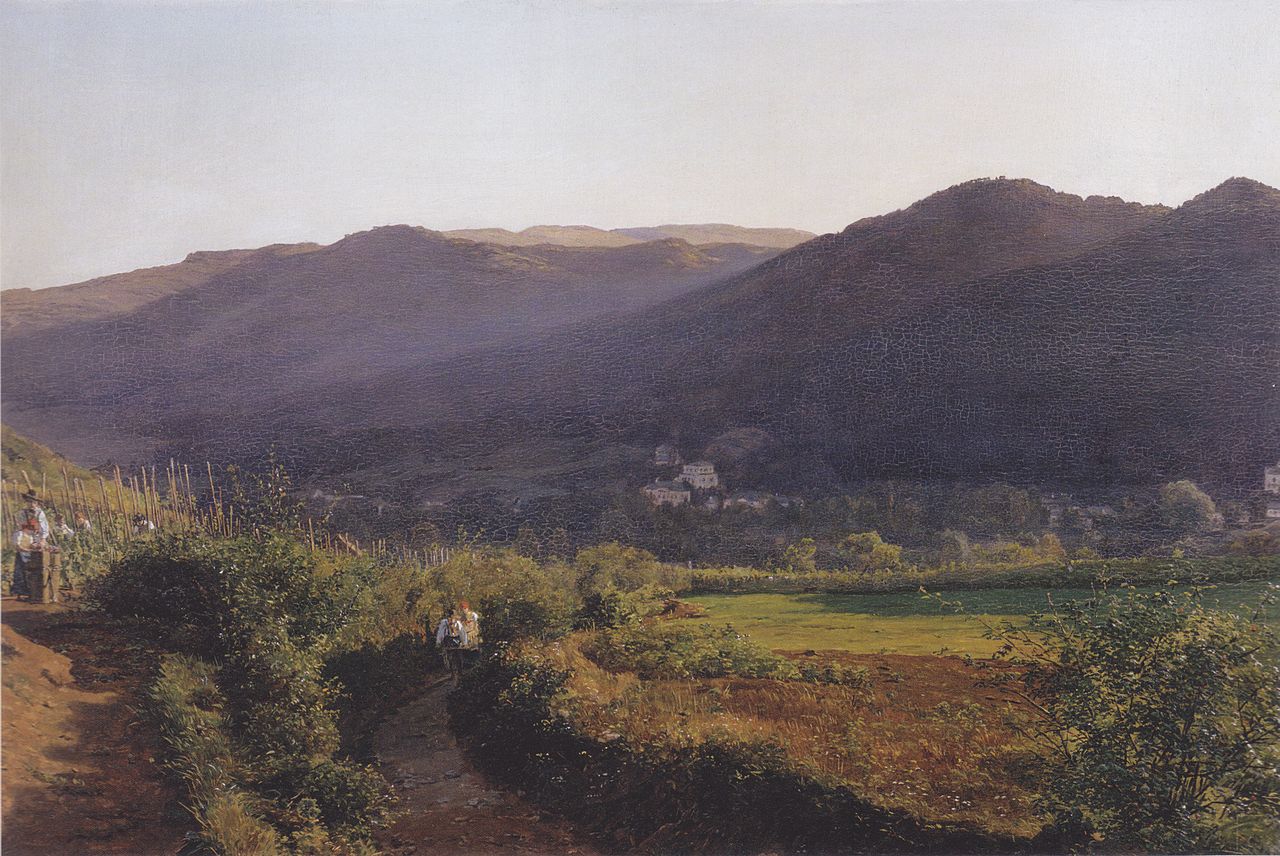This landscape painting captures a serene countryside scene in late afternoon. In the foreground, a rich brown field stretches out, intersected by a dirt path. The field is flanked by patches of green shrubbery and small clusters of dark green trees predominantly situated on the left. Scattered across the field, small figures, possibly farmers, are engaged in their tasks, adding a touch of life to the tranquil setting. 

Midway through the composition, a few white houses with gabled roofs nestle at the base of gently sweeping mountains. The mountains themselves are a mix of brown and purple hues, with hints of fog settling in the valleys, adding to the scene's dreamy and misty ambiance. 

In the backdrop, the mountains rise gracefully towards a sky that transitions from a hazy white at the horizon to a grayish blue higher up, suggesting an overcast day with the soft glow of sunlight filtering through the clouds. The overall mood of the painting is calm and idyllic, capturing the quiet beauty of rural life against a majestic natural terrain.